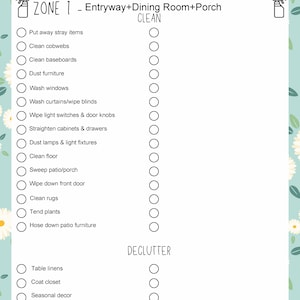A photograph captures a computer screen displaying a detailed cleaning checklist labeled "Zone 1: Entryway, Dining Room, and Porch." The list includes various cleaning tasks, each preceded by a checkable circle. Tasks range from "put away stray items," "clean cobwebs," "clean baseboards," "dust furniture," "wash windows," "wash curtains," "wipe blinds," and "wipe light switches and doorknobs," to "straighten cabinets and drawers," "dust lamps and light fixtures," "clean floors," "sweep patio porch," "wipe down front door," "clean rugs," "tend plants," and "hose down patio furniture." The checklist likely serves as a communication tool for household staff, allowing them to mark tasks as completed. Additionally, the screen features a section titled "Declutter," listing "table linens," "coat closet," and "seasonal decor," although this section is partially cut off in the photo. The image provides a clear, organized view of household cleaning priorities within specific zones.